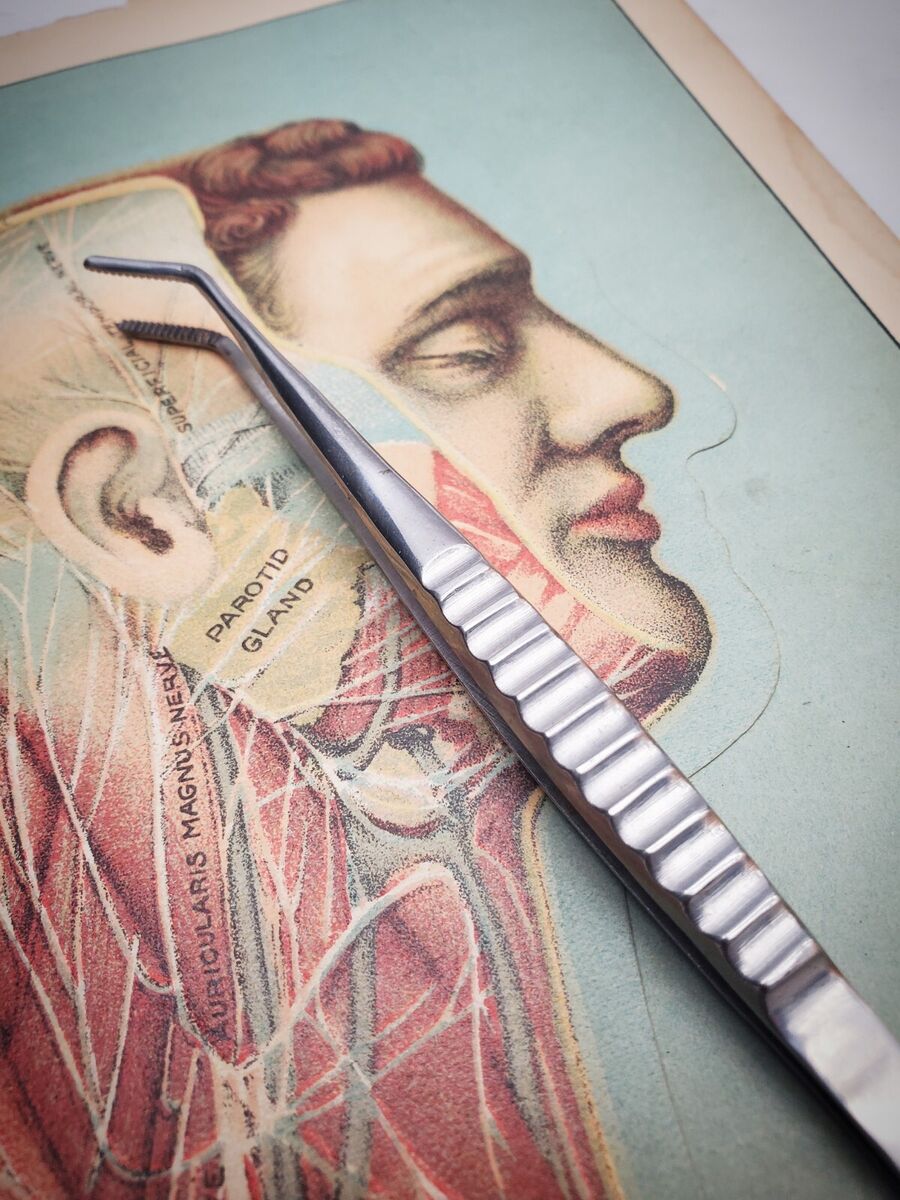The image appears to be an illustration from an antique medical book, possibly framed for display. The picture features a detailed anatomical drawing of a man's right profile. The man is light-skinned with curly red hair and closed eyes. His facial skin has been meticulously cut away to expose underlying structures, including the skull, veins, and nerves. The visible ear retains its flesh but is intricately depicted with veins and additional nerves extending from the cheek down to the neck and upper chest.

The background of the image is a light slate blue or slate gray, providing a subtle contrast to the detailed anatomical features. The entire illustration is encased in a wooden frame. Additionally, a silver instrument, likely a pair of tweezers, is placed on top of the frame, adding a contextual touch representative of medical examination or display. In the backdrop, there appears to be a gray table, enhancing the overall sense of an academic or clinical setting.